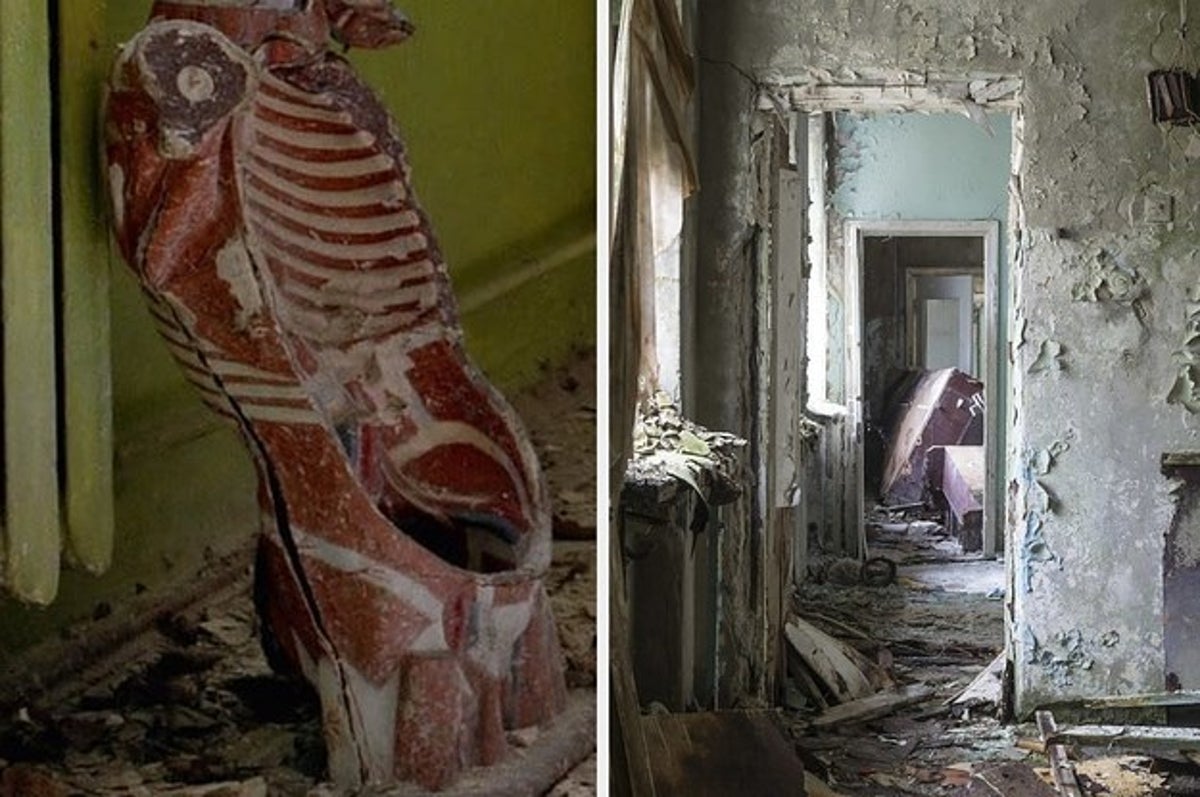The image is a collage of two photographs, likely taken in the same abandoned building. On the right, a rundown white-painted building is visible with peeling paint and decayed walls. Through an open doorway devoid of a door, we see into a hallway leading to what appears to be a bedroom, where everything is in disarray; a mattress is turned on its side among various debris scattered on the decayed floor. The room features a window on the left wall, allowing daylight to seep through and highlighting old, decrepit curtains. 

On the left side of the collage, there is an anatomical model resembling a human torso without arms or legs, exposing muscle and bone structures in red and white. The model, standing amidst debris on a lime-green backdrop, depicts a cut-open ribcage, showing detailed inner cartilage and skeletal elements. The scene conveys a sense of decay and abandonment, linking the two images through their shared depiction of desolation and deterioration.